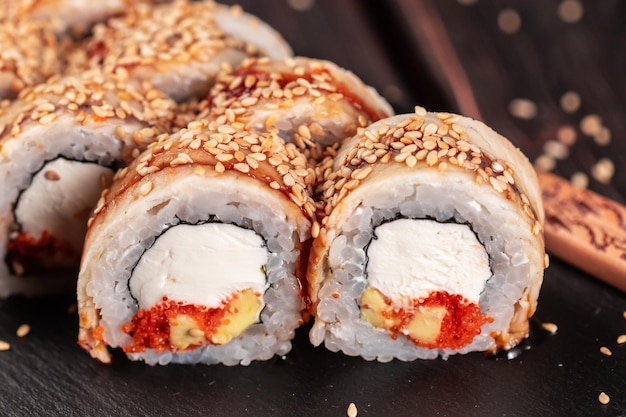The close-up photograph showcases an array of visually appealing sushi rolls artfully arranged on a black-painted wooden surface. The horizontally aligned rectangular image offers a detailed view, particularly focused on two prominent rolls in the foreground, while additional rolls recede into a blur toward the upper left. Each sushi roll features a rice exterior generously adorned with a myriad of tiny sesame seeds. The rolls boast a creamy white center that could be either cream cheese or sour cream, accompanied by a speckling of red sauce and yellow toppings, likely fish roe. The top of the rolls is garnished with what appears to be shaved almonds, giving them a crusted brown appearance. Loose seeds are scattered around, enhancing the texture and appeal of the dish.